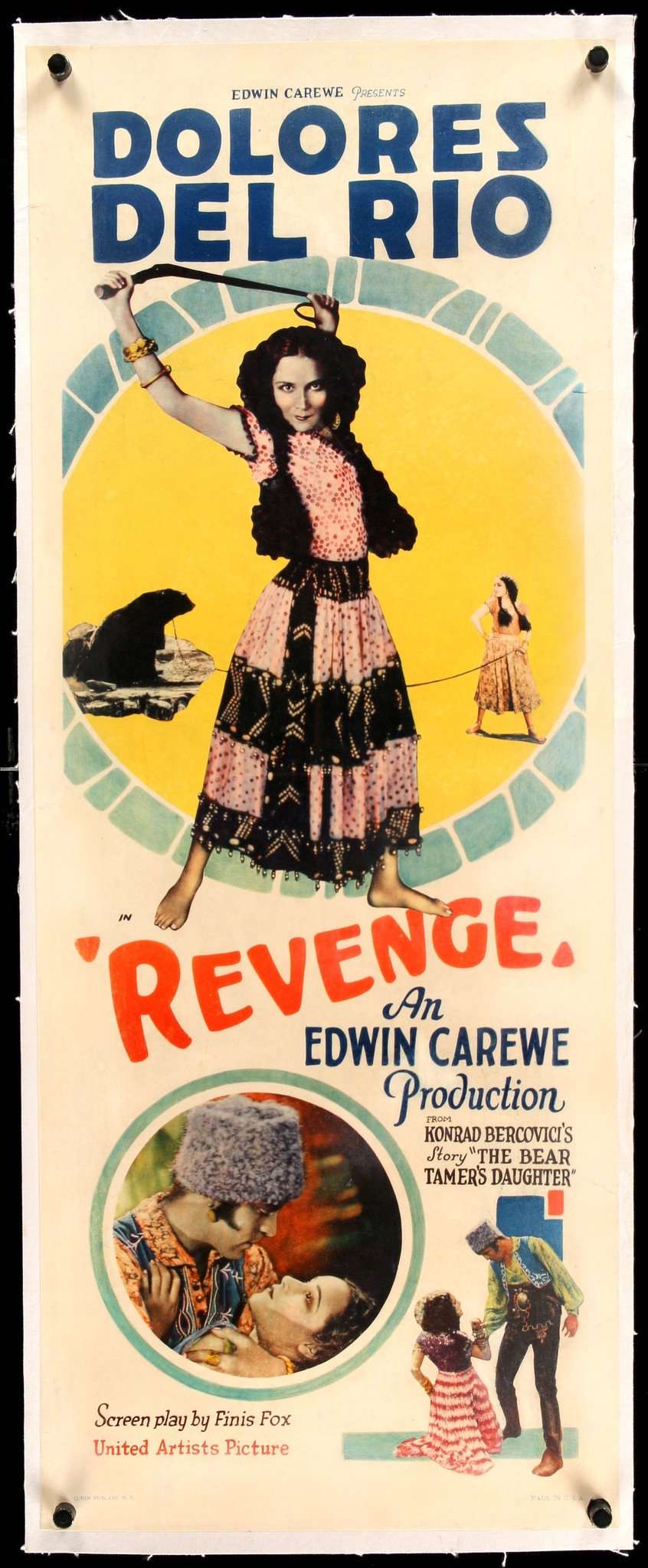The vintage movie poster titled "Revenge," produced by Edwin Carravee and based on Conrad Bercovici's story "The Bear Tamer's Daughter," prominently features the renowned actress Dolores Del Rio. The poster, with slightly tattered edges and mounted on a black surface using black thumbtacks, boasts a striking design. The background of the poster is light orange, and it is printed on white paper. At the top, large blue letters announce "Edwin Carravee presents Dolores Del Rio." Dolores is depicted in the center wearing a striking pink and black costume, her hands raised, gripping a whip. Beside her, a woman is seen holding a rope tethered to a black bear. Below this central image, bold red wavy text reads "Revenge," followed by smaller blue text detailing "an Edwin Carraway Production." At the bottom of the poster, there are two smaller images: one shows a man and woman embracing, with the woman's image encircled by a gray-bordered circle. This visually rich and detailed poster captures the dramatic essence of the film.